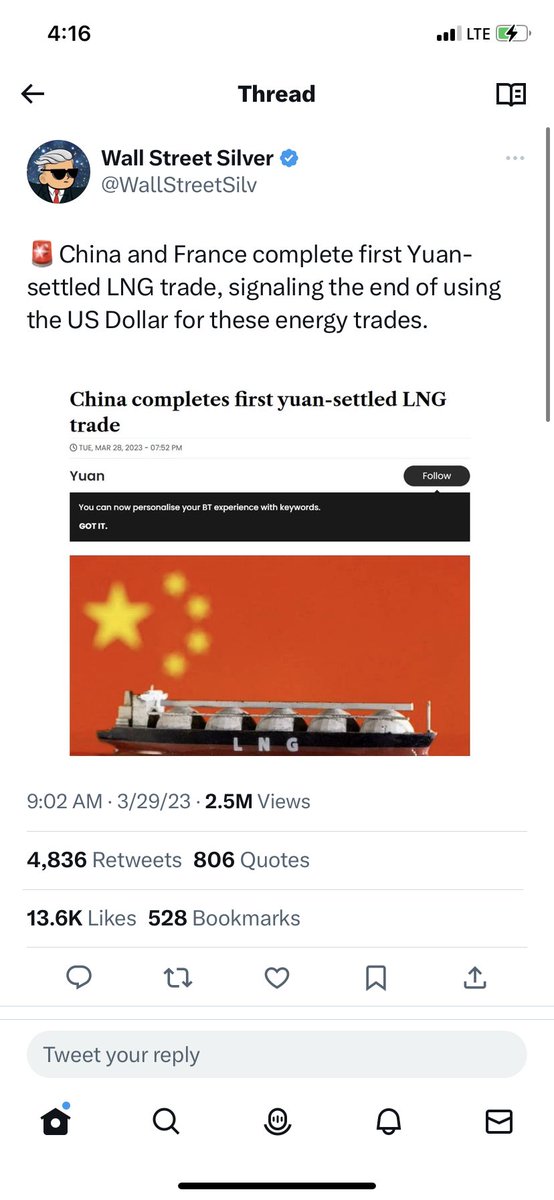**Image Caption:**

At the top of the screen, the status bar displays '4:16,' with three out of four bars for LTE signal strength, a half-full battery with a lightning bolt indicating charging, a back arrow, a thread icon, and a book icon. The main focus is a silhouette of a man with slicked-back gray hair, glasses, and a suit, captioned "Wall Street Silver."

The text next to the silhouette reads: "Wall Street Silk" and further down, a headline says, "China and France Complete First Yuan-Settled LNG Trade, Signaling the End of Using the US Dollar for These Energy Trades." 

Another line emphasizes, "China Completes First Yuan-Settled LNG Trade."

A follow-up prompt advises, "You can now personalize your IT experience with keywords."

To the side of these texts, there is a red flag featuring a yellow star and three surrounding yellow dots, alongside a scale holding five silver balls, labeled "LNG."

Below, the timestamp reads "9:02 a.m., 3/29/23," with engagement metrics: 2.5M views, 4,836 retweets, 806 quotes, 13.6K likes, and 528 bookmarks. Social media engagement icons are visible: a chat icon, two swirling arrows, a heart, a ribbon, and an upload icon.

At the bottom, an input field prompts users to "Tweet Your Reply."

The navigation bar at the bottom shows icons of a house with a blue dot, a search icon, a microphone, a bell, and an envelope. The screen is divided by a black line.